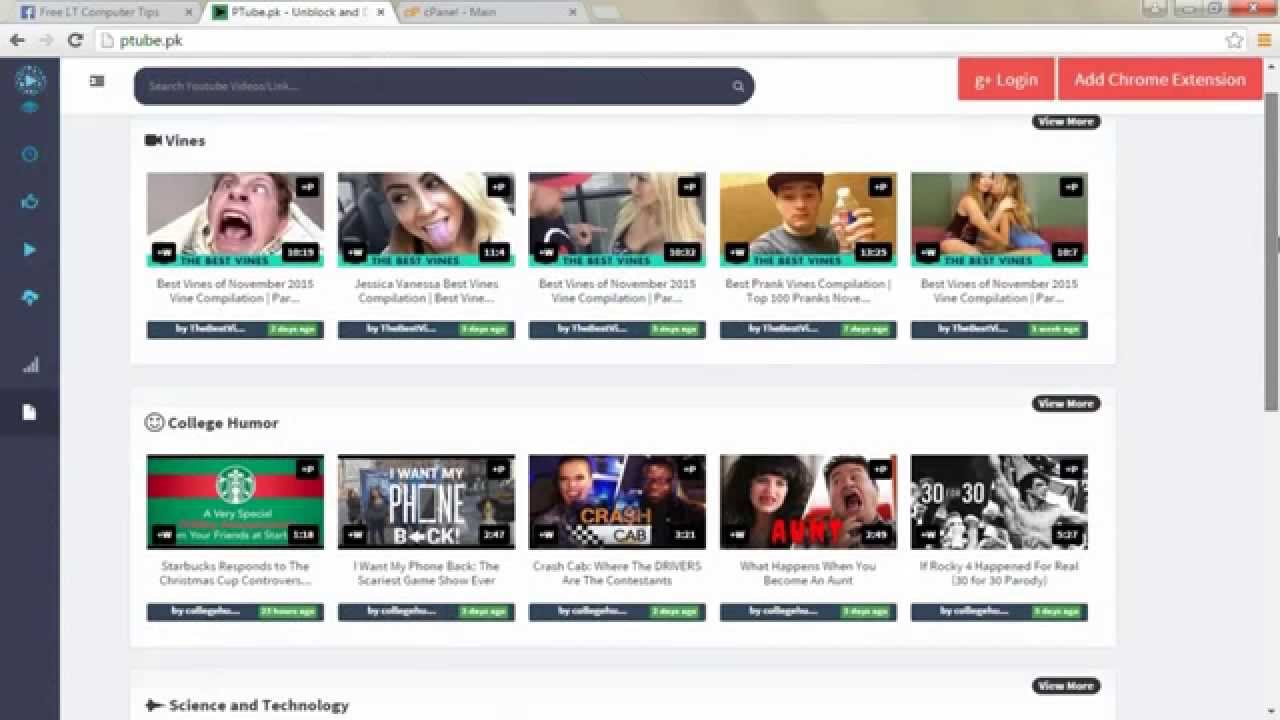The image depicts a web browser window with three open tabs, focusing on the center tab. The URL in the address bar reads "p2.pk." On the left side of the address bar, there are several indistinct buttons including a recognizable play button. Adjacent to the address bar on the right is a search bar. The top of the window features a prominent red "Log In" button, accompanied by a larger red button labeled "Add Chrome Extension." Directly below, an icon of a video camera labeled "Vines" is visible, followed by five video thumbnails, each accompanied by a description in a green box. Further down the page, there is a section titled "College Humor" which also contains five video thumbnails with corresponding descriptions. The bottom section features "Science and Technology" and lists related video thumbnails and their descriptions.